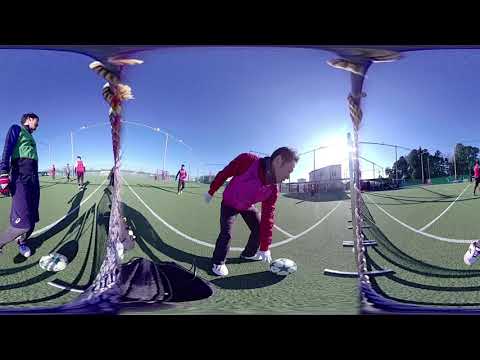A vibrant, sunny day captures a dynamic soccer practice on a field. The image, seemingly taken with a fisheye lens or a camera creating a triptych effect, shows a bustling scene under a blue sky. Central is a man bending down to pick up a soccer ball with purple accents while wearing a pink jacket, black sweatpants, and white shoes. To the left, another player, standing with a volleyball in front of them, dons purple shorts and red gloves, casually observing the field. Behind these figures, other players in similar pink and black athletic gear are scattered. The right side features a building amidst various trees, adding depth to the background. The overall bright and clear atmospheric conditions suggest a perfect day for outdoor sports activities.